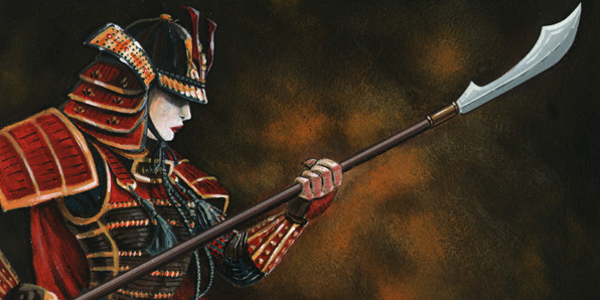The image is a rectangular illustration, about twice as wide as it is tall, depicting a female warrior resembling a samurai or shogun. She wears elaborate, traditional Japanese armor composed of black and red plates adorned with gold gilding. Her helmet features multiple plates extending down the back of her head and a tip that descends over her brow and bridge of her nose, obscuring her eyes. The helmet is richly detailed in red, orange, and black. Her face is painted white with striking red lipstick.

Her upper body is protected by a black chest piece also featuring gold details, and black tassels hang from straps on her shoulders. She grips a long weapon, presumably a halberd, with both hands. Her left hand is positioned near the front of the handle, extending forward and up, while her right hand is at the base, closer to her side.

The background behind her consists of a cloudy, smoky blend of amber, orange, and black hues, evoking the imagery of a battlefield.